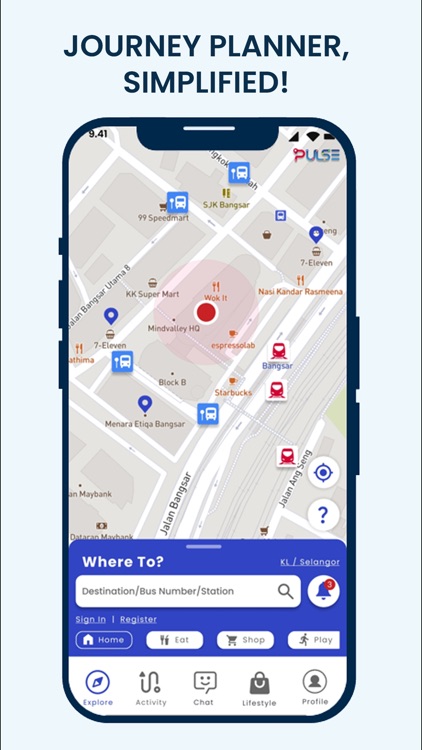Rectangular Image with Light Blue Background Featuring a Smart Travel Planner Interface:

This rectangular image displays a light blue background, featuring the interface of a journey planner application. Centered at the top in dark print, the text "Journey Planner Simplified" prominently stands out. Below this headline, a smartphone screen dominates the imagery, giving a detailed representation of the app's functionalities.

In the upper sections of the phone's screen, the time "9:41" is displayed on the left, while typical status icons for cellular and wireless connections appear on the right. Below these, on the right-hand side, the name "Pulse" is visible.

The main focus within the smartphone screen is a digital map covering most of the display. This map showcases various labeled points of interest, including "KK Supermart," "Block B," and "7-11." Multiple blue pins mark different locations on the map, and a specific point is highlighted with a red circle. The map also features illustrations of red trains and a blue and white bus at a bus stop, symbolizing transportation options.

Towards the bottom of the map, "Where To" text is displayed above a search box which is labeled with "destination/bus number/station." Adjacent to this search box, a white circle contains a blue bell icon with the number '3' inside a red circle, potentially signifying notifications.

Underneath the map, users are given the options to "Sign In" or "Register," followed by a home button and additional icons labeled "Eat," "Shop," and "Play." At the very bottom of the phone screen, a set of navigation icons is present for "Explore," "Activity," "Chat," "Lifestyle," and "Profile."